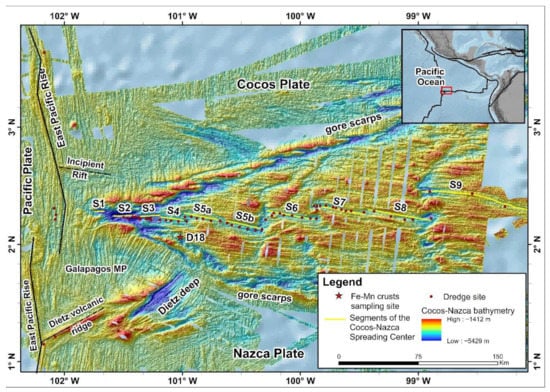This is a highly detailed, horizontally oriented topographic map depicting the Cocos and Nazca tectonic plates, their interactions, and various geological features in the Pacific Ocean. The main map is colorful, using hues from red to blue to signify different elevations, with red indicating higher elevations and blue indicating lower. It includes notable labels such as Cocos Plate, Nazca Plate, East Pacific Rise, Dietz Volcanic Ridge, and several scarps.

In the upper right corner, there is an inset showing the location of the mapped area within the Pacific Ocean, highlighted by a red rectangle. Coordinates frame the map, ranging from 99 to 102 degrees west longitude and from 1 to 3 degrees north latitude.

The bottom right corner houses a detailed legend in a white box. The legend explains the symbols used: stars for FE-MN Crust Sampling Sites, dots for dredge sites, and yellow lines for segments of the Cocos-Nazca Spreading Center. It also outlines the bathymetric gradient, ranging from high elevations at 1412 meters to low areas at 5429 meters below sea level. The map effectively combines topographical and geological information to provide an intricate view of this underwater region.